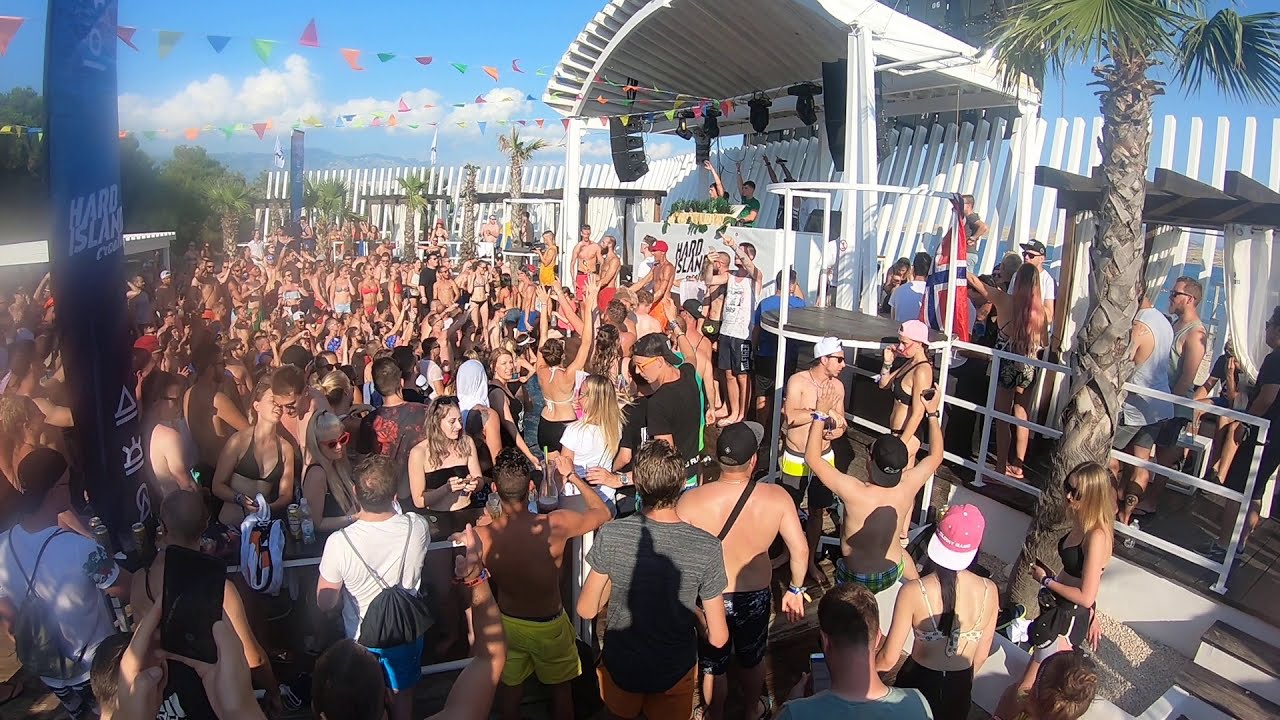This is a vibrant landscape photograph capturing an outdoor festival teeming with a large crowd of people, likely in their 20s, dressed in summer or beach attire. Men can be seen shirtless, while women are clad in bathing suit tops or tank tops. Many attendees wear sunglasses, hats, and backpacks, creating a festive and carefree atmosphere indicative of a warm climate, possibly a spring break event. The crowd, composed of hundreds of revelers, is primarily facing a stage off to the right, where a DJ or performer in a white shirt, black shorts, and a red baseball hat is entertaining the masses under a white pergola. The background features blue skies adorned with white clouds, colorful flags in shades of purple, orange, yellow, and blue, as well as palm trees that add to the tropical feel. A blue sign on the left side of the image prominently displays "Hard Island." A white fence surrounds the area, enhancing the scene's sense of an organized but energetic celebration.